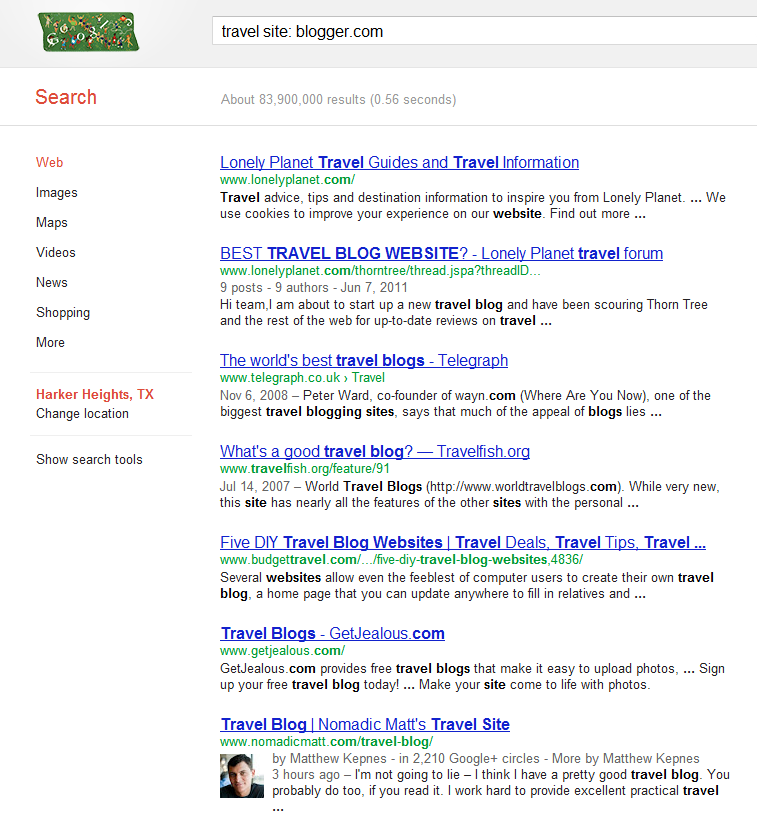The image depicts a search results screen, likely from a travel-related website. The upper portion of the screen features a gray border. In the upper left-hand corner, there is a green rectangle adorned with various colorful graphics. Adjacent to this, on the right, is a search bar displaying the text "TravelSiteBlogger.com." 

Moving down, a prominent white bar contains the word "Search" in red, with an indication to the right showing "About 80,900,000 results." On the left side, there is a vertical menu listing options such as "Web," "Images," "Maps," "Videos," "News," "Shopping," and more, with "Web" highlighted in red. Below this is the location "Parker Heights, Texas" in red text, followed by a "Change Location" option and a "Show Search Tools" button.

On the right side, the first search result is titled "Lonely Planet Travel Guides and Travel Information" in blue with an underline, attributed to "LonelyPlanet.com." The second result, "Best Travel Blog Website, Lonely Planet Travel Forum," follows a similar format with a title in blue and an underlining. 

The third result is "The World's Best Travel Blogs" from Telegraph, also in blue with an underline. The fourth result, "What's a Good Travel Blog from TravelFish.org," includes a description underneath. Subsequent results are "5 DIY Travel Blog Websites, Travel Deals, Travel Tips" with additional information, "Travel Blogs, GetJealous.com" with a description underneath, and finally "Travel Blog, Nomadic Matt's Travel Site," also accompanied by a description.